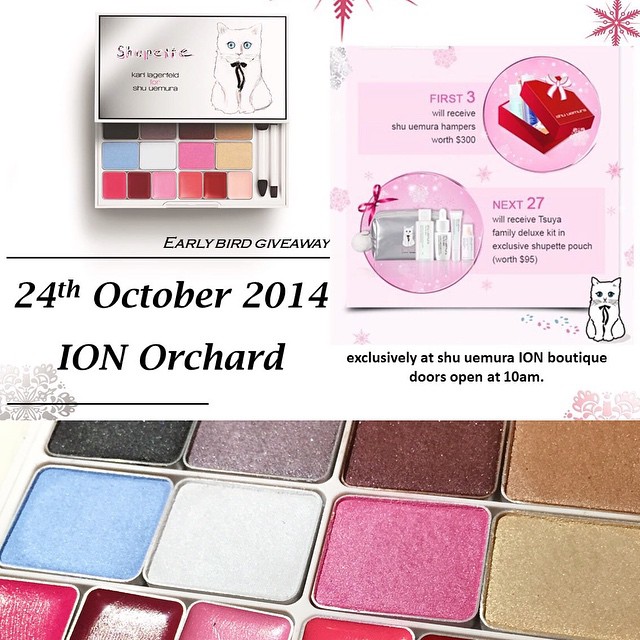The image appears to be an advertisement for a make-up sale, specifically a giveaway event hosted by Shu Uemura. Dominating the top section of the page is a white eyeshadow compact adorned with a cat illustration; the cat has wide blue eyes and wears a long black ribbon around its neck. This compact is identified as the "Shupet Palette," a collaboration between Karl Lagerfeld and Shu Uemura. To the left of the compact, the text "Early Bird Giveaway" is prominently displayed in black. Below this sits a black line, under which the date "24th October 2014" is mentioned along with the location "ION Space Orchard" in bold capital letters. Further right, in smaller print, it specifies "Exclusively at Shu Uemura ION," followed by "Doors Open at 10 a.m."

The palette itself features neutral browns, blue, white, pink, and yellow eyeshadows, alongside small sponge tip applicators, and blushes in various shades of pink and red. To the right of the main image, a pink box contains details of the giveaway prizes. The top section shows a red box and text indicating that the "first three" winners will receive Shu Uemura hampers worth $300. Below, further details state that the "next 27" winners will receive a Tsuya Family Deluxe Kit and an exclusive Shupet pouch worth $95. Adjacent to this text, a silver pouch bearing the same cat illustration is displayed, along with various bottles and tubes.

The central section of the image is brought into focus with another depiction of the event date and location, again highlighting the exclusivity at Shu Uemura ION Boutique with doors opening at 10 a.m. The image concludes with a close-up of the make-up compact, showcasing the textures and vibrant colors of the eyeshadows for a detailed view of the product.